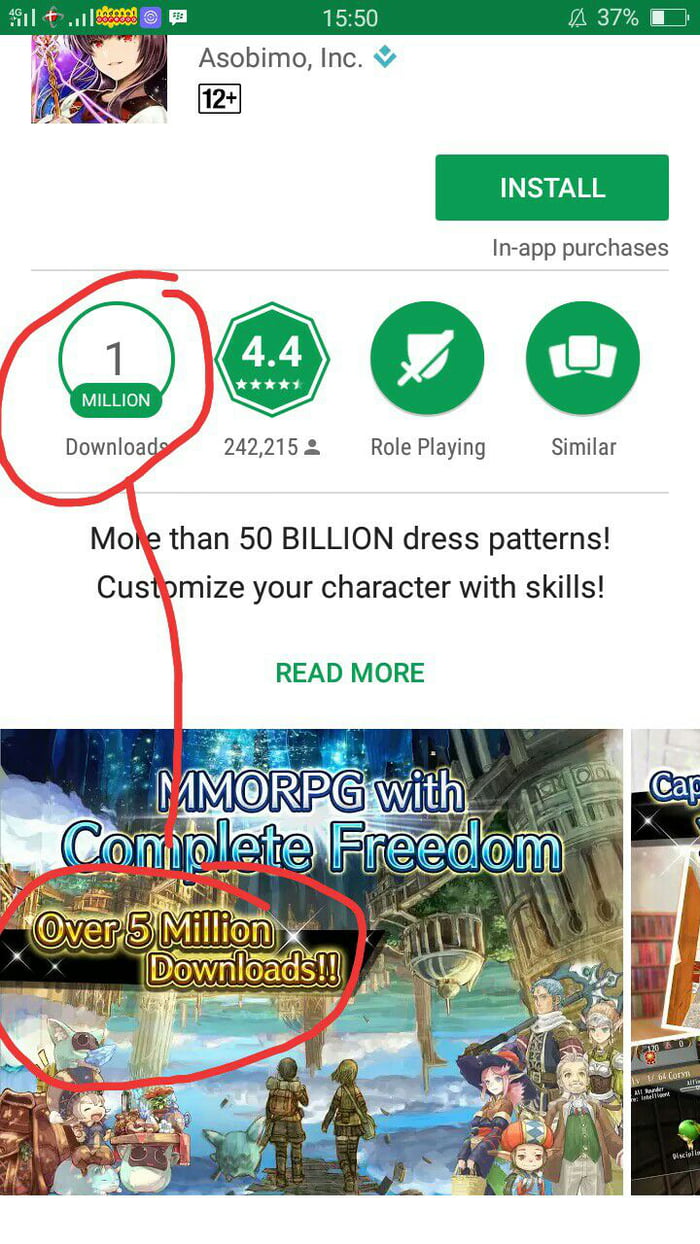This image appears to be a screenshot taken on an Android phone of a Google Play Store page. At the very top, there's a green status bar displaying a battery level of 37%, the time as 15:50, and indicators for Wi-Fi and network signal strength. There are also a few icons suggesting the presence of messages or notifications.

The focus of the image is on a game, although the game's name is partially obscured. A fragment of an anime-style cartoon face is visible, hinting at the game's visual style. The publisher is identified as ASOBIMO, Inc., and the game has a 12+ age rating. A green "Install" button is prominently displayed, with a note below it indicating that the game includes in-app purchases.

Further down, the image is annotated with four small icons arranged in a row. The first icon, encircled in red, states "1 million downloads." The second displays a rating of "4.4 stars," the third features a shield and sword icon denoting the game as "Role Playing," and the fourth simply says "Similar."

A red line has been drawn from the "1 million downloads" icon to another piece of text circled at the bottom of the screen, which reads "over 5 million downloads." This suggests a discrepancy between the two download figures, possibly due to differences in counting downloads across various platforms.

At the bottom of the image, additional text reads, "MMORPG with complete freedom - over 5 million downloads," providing further context about the game. The annotation highlights a potential inconsistency in the download statistics presented by the publisher versus what is shown on the Google Play Store.